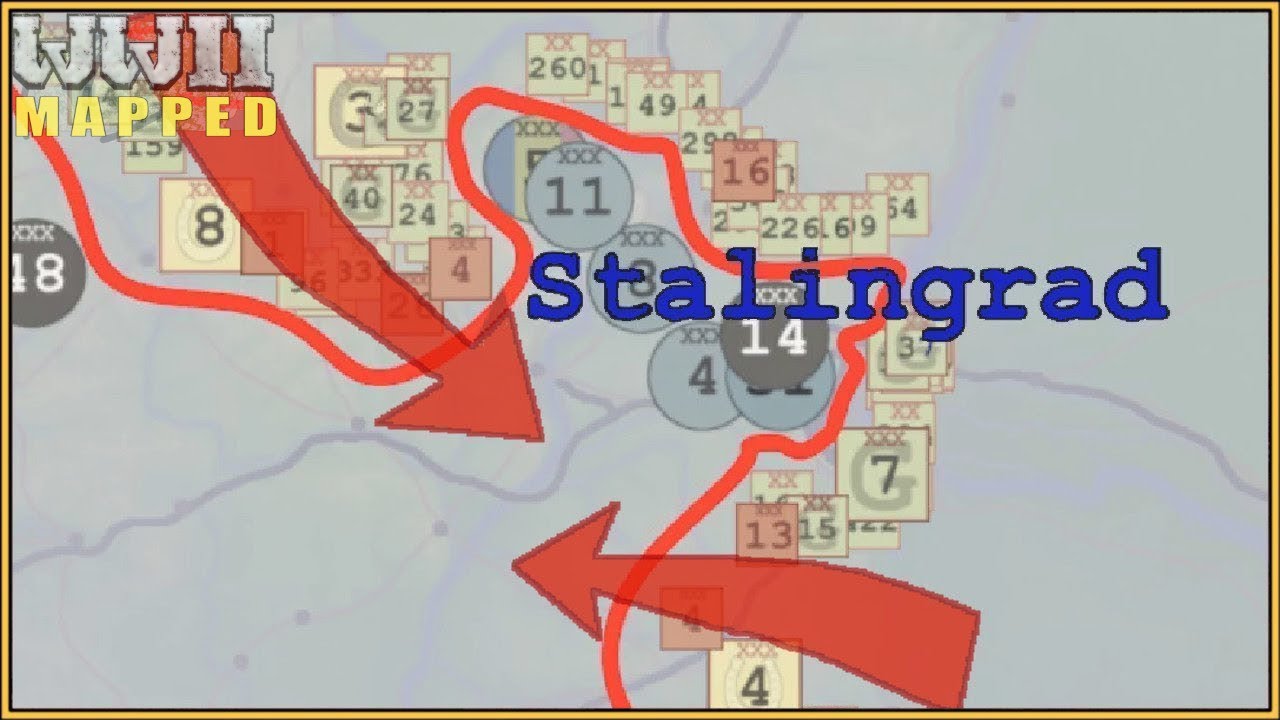The image is a detailed WWII map characterized by numerous visual elements and annotations. Dominating the map are large red arrows indicating the movement of soldier fronts, one descending from the top and the other emerging from the right, converging offset to the bottom left of the center. The map's background is a light greyish-blue with a yellow border framing it. In the top left corner, bold white text reads "WWII," and below it, "MAPPED" in uppercase yellow letters. Central and slightly to the right, large blue text prominently labels "Stalingrad." Scattered across the map are multiple beige-yellow squares marked with various numbers, including some with red backgrounds and multiple black Xs (such as 16, 4, and 13). These squares appear to indicate different positions or units. Two red Xs and red outlines highlight some specific squares. A red squiggly line loops from the top left around the middle and descends to the bottom, likely symbolizing a river. Additional grey circles with numbers and Xs are interspersed, adding to the intricate detailing of the map. The overall depiction suggests strategic movements and key locations pertinent to World War II.